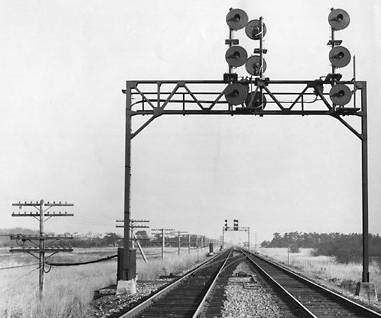This black and white image depicts a long-range view of side-by-side railroad tracks extending all the way to the horizon, where they appear to converge. Between the two sets of tracks is a curved connector track, allowing trains to move from one track to the other. In the foreground, two tall posts support a horizontal bar, from which hang three traffic signal lights, likely for conducting train traffic. The tracks themselves are bordered by gravel, with fields of short grass and several electrical poles stretching into the distance, one on the left side of the tracks and three on the right. The scene is enveloped in a gray, cloudy sky, lending an overall somber tone to the image.